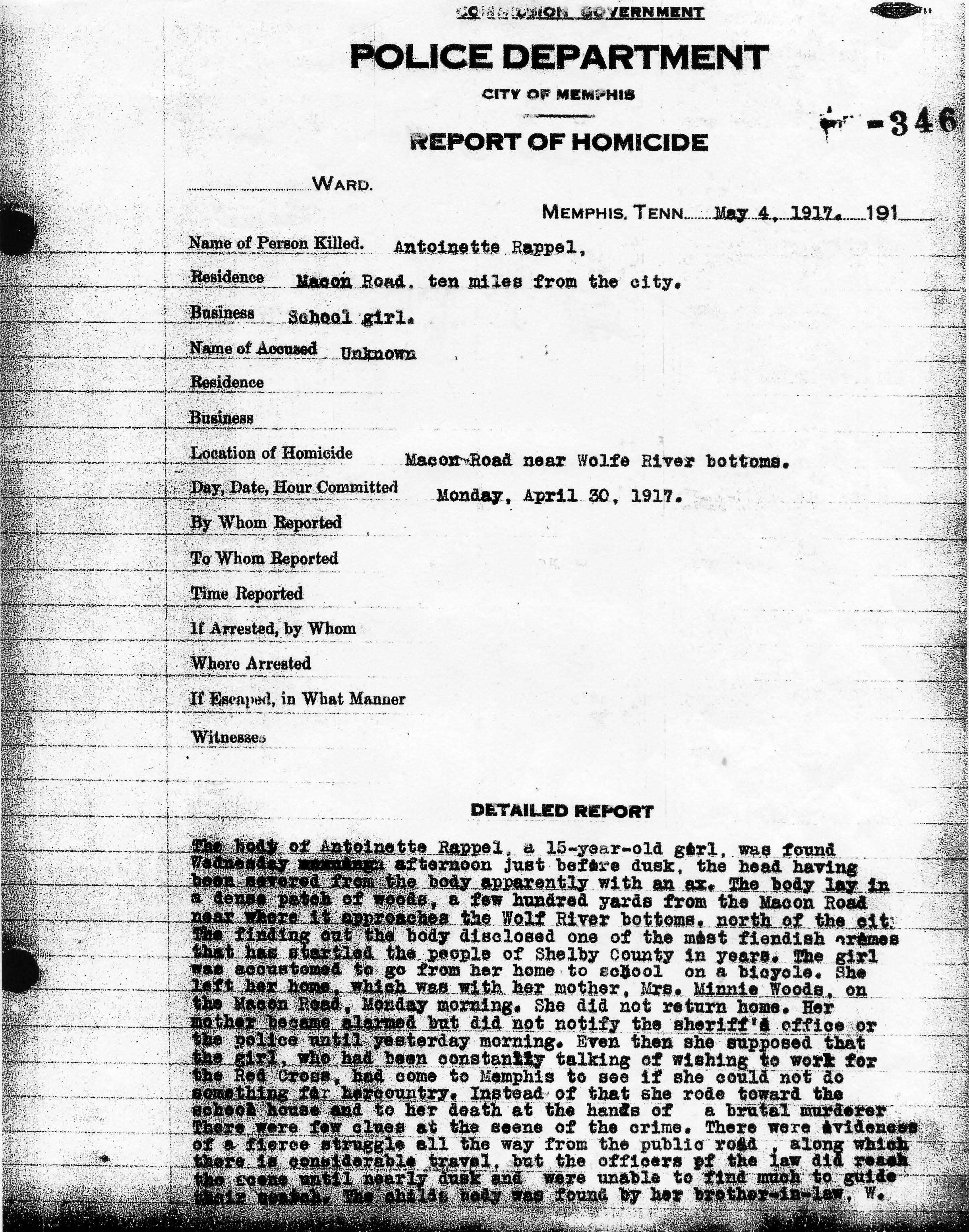The image appears to be a scanned copy of an aged police report printed on lined notebook paper, visible through the paper's distinctive binder holes and shadowed edges possibly due to multiple photocopying or faxing. This black-and-white document, dated May 4th, 1917, by the Memphis Police Department, is titled "Report of Homicide" with the case number 346. The report details the homicide of Antoinette Rappel, a 15-year-old schoolgirl residing 10 miles from Memphis, found murdered near the Wolf River Bottoms on April 30th, 1917. Antoinette had left home for school on her bicycle but never returned, and her body was discovered later, showing evidence of a struggle and gruesome injuries inflicted with an ax. The name of the accused remains unknown, and the report contains a difficult-to-read paragraph detailing the circumstances around the crime, likely muddied due to the report’s repeated scanning and copying over the years.